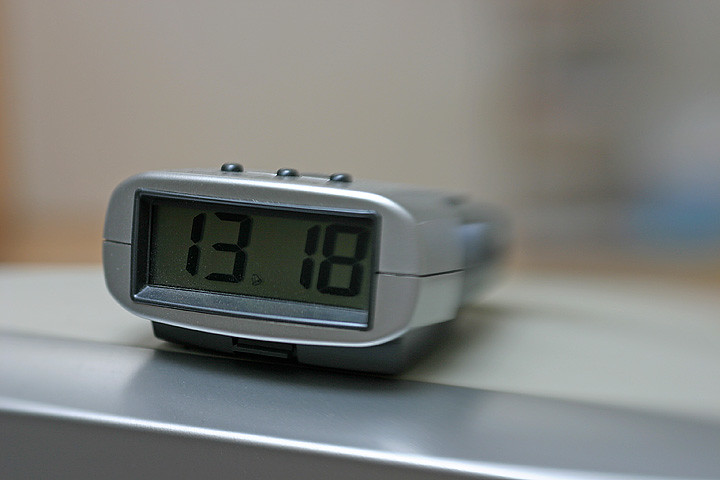This is a close-up photograph taken indoors with a regular camera, focusing on a small, silver travel alarm clock positioned centrally. The clock features a front LCD screen displaying the time "1318" in black digital numbers against a light gray background. The top of the alarm clock is equipped with three deep gray buttons serving as controls, and its lower section is of a slightly dark gray hue. The clock is resting on a light gray dresser with a metal base. The background is intentionally blurred, providing an indistinct view of a peach-toned wall and possibly a brown or beige shelf displaying a few items, including a noticeable blue object and a tiny strip of chrome running horizontally.